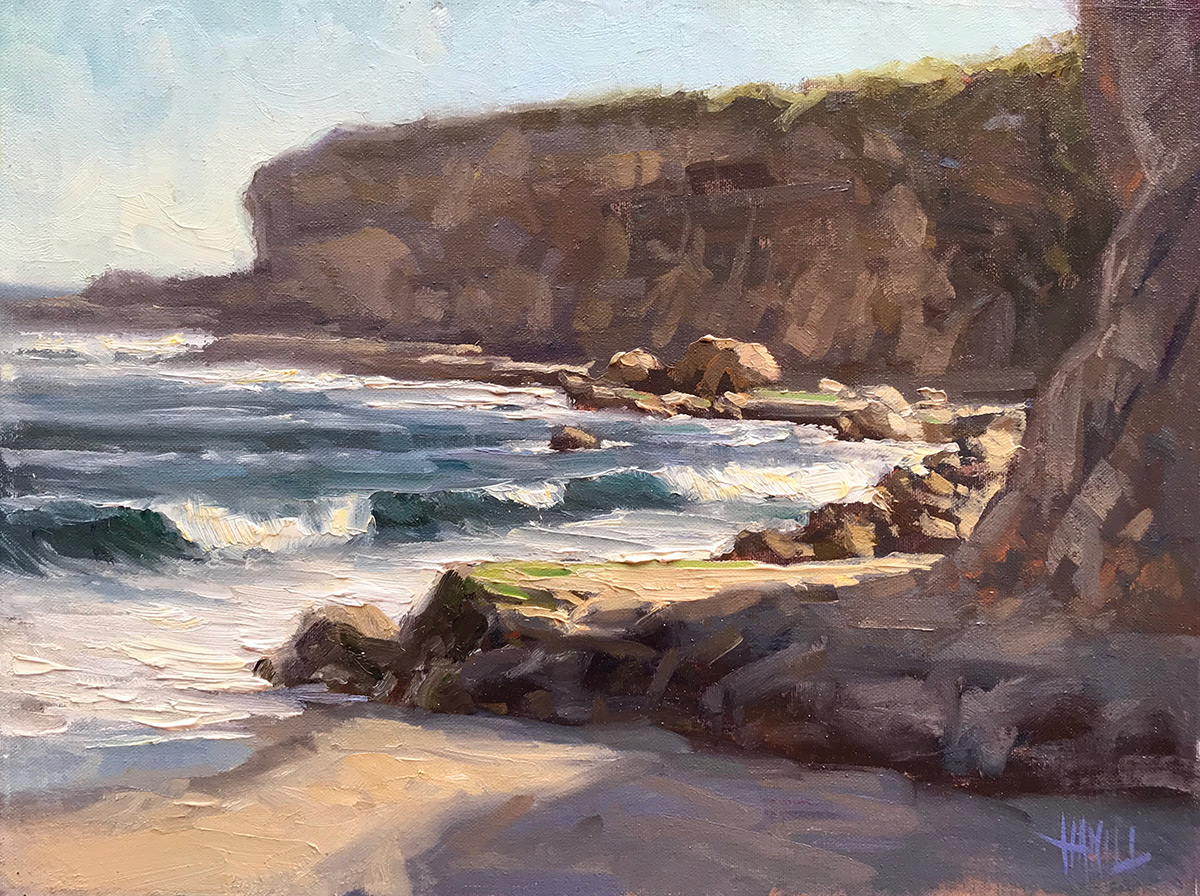This artwork is a vertically aligned rectangular painting, likely an oil painting given the thickly textured white areas of water near the beach. The scene is an outdoor beach cove during the daytime, capturing a dramatic and rugged coastal landscape. The upper portion of the painting depicts a sky with a blend of white and light blue hues. Dominating the center and extending to the right is a towering cliff adorned with medium to dark brown shades and a touch of green at the top, suggesting grass. This cliff descends into the foreground, where it meets a narrow, flat, sandy shoreline. The sand is primarily medium brown, accented with darker brown and gray shadows cast by the rock formation. On the left side, the painting features dynamic ocean waves rendered in dark blue and white, crashing into the rocks scattered along the shore. Several loose rocks are visible near the shoreline. In the bottom right corner, there's a handwritten signature, possibly the artist's initials, starting with an H and written in purple, though it is difficult to decipher fully.